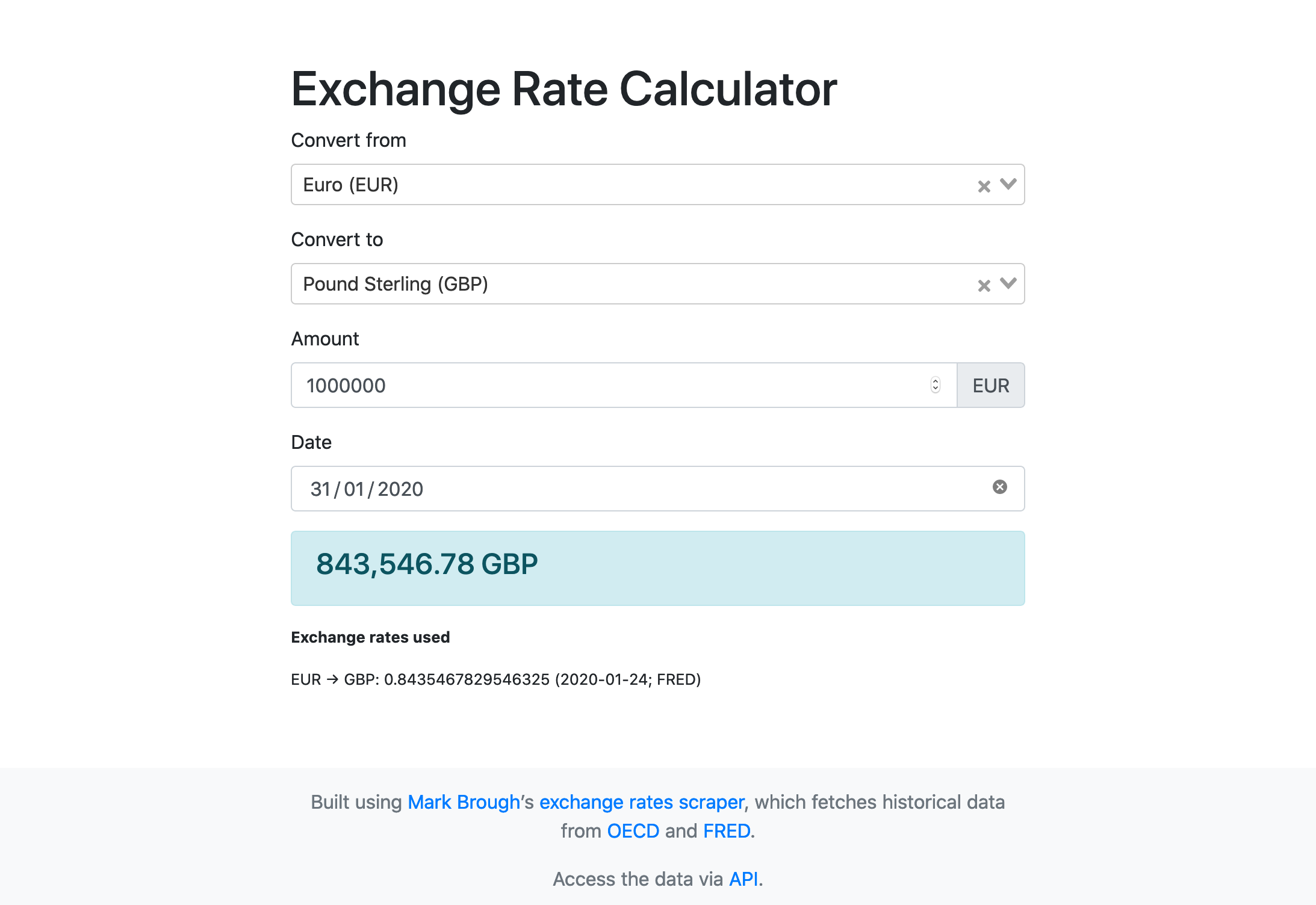**Descriptive Caption:**
The website showcases an Exchange Rate Calculator application with a clean, minimalist design featuring a white background and black text. At the top of the webpage, a prominent header reads "Exchange Rate Calculator." Below it, two sections prompt the user to convert currencies: "Convert from Euros" and "Convert to Pounds Sterling." The input amount is specified as "100,000 Euros."

A notable feature is a small, blue rectangular banner positioned in the lower section of the page, displaying the converted amount: "843,546.78 GBP." Detailing the conversion rate, the webpage states that the exchange rate used is 0.8435 Euros to GBP. Additionally, the date of the conversion is marked as "31.01.2020."

At the bottom of the page, a technical footnote acknowledges the tools used to build the calculator: "Built using Mark Burroughs Exchange Rate Scraper which fetches historic data from OECD and FRED. Access the data via API." The application merges historical data sourcing and real-time API access to offer precise currency conversion results.